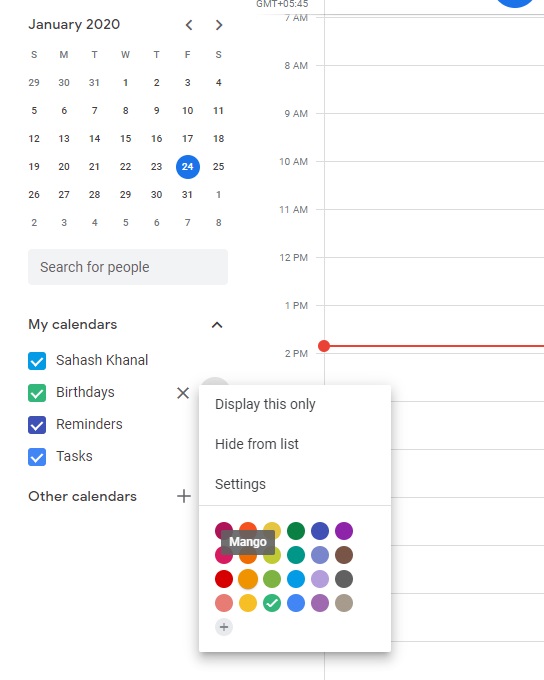Displaying a detailed image of a digital calendar for January 2020, the left side prominently shows a monthly grid with black numbers on a white background. The date "24" is highlighted with a blue circle. Below the calendar, there are navigational options such as "Search for People," and a list labeled "My Calendars" features entries including "Saha Sh," "Kanaan al," alongside categories like "Birthdays," "Reminders," "Tasks," and "Other Calendars."

On the right side of the image, there is a daily agenda view with hourly slots listed from 7 a.m. to 2 p.m. A red line extends horizontally just above the 2 p.m. slot, originating from a small red dot. A contextual pop-up menu provides options including "Display this only," "Hide from list," and "Settings," alongside a color palette featuring red, orange, yellow, green, blue, purple, brown, and black squares.

Additionally, a black rectangle labeled "Mango" in white text obstructs part of the agenda view, concealing the times below it. At the top of the image, above the 7 a.m. slot, there's a time zone mention "GMT+05:45" partially overlapped by a blue circle, of which only the bottom sliver is visible.